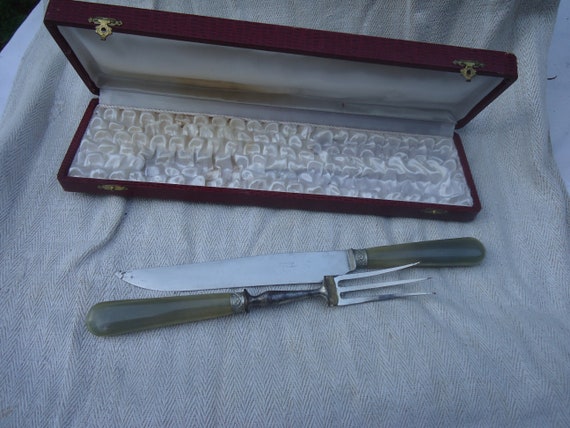This is an image of a collectible carving set consisting of a fork and a knife with jade-like dark green handles and silver tips, elegantly arranged on an off-white cloth. The fork, positioned at the very bottom with its tines facing downwards, has a sleek and simple design. Directly above it, the matching knife features a similar dark green handle, resembling jade, and a polished silver blade. Above these utensils is an old, distinguished wooden case with brass or copper clasps. The dark-stained case, which appears sturdy and well-crafted, has a soft white, velvet-like interior padding to cradle the utensils securely. The image is rather dark, casting the items in shadow, lending the scene an antique, almost mystical quality.